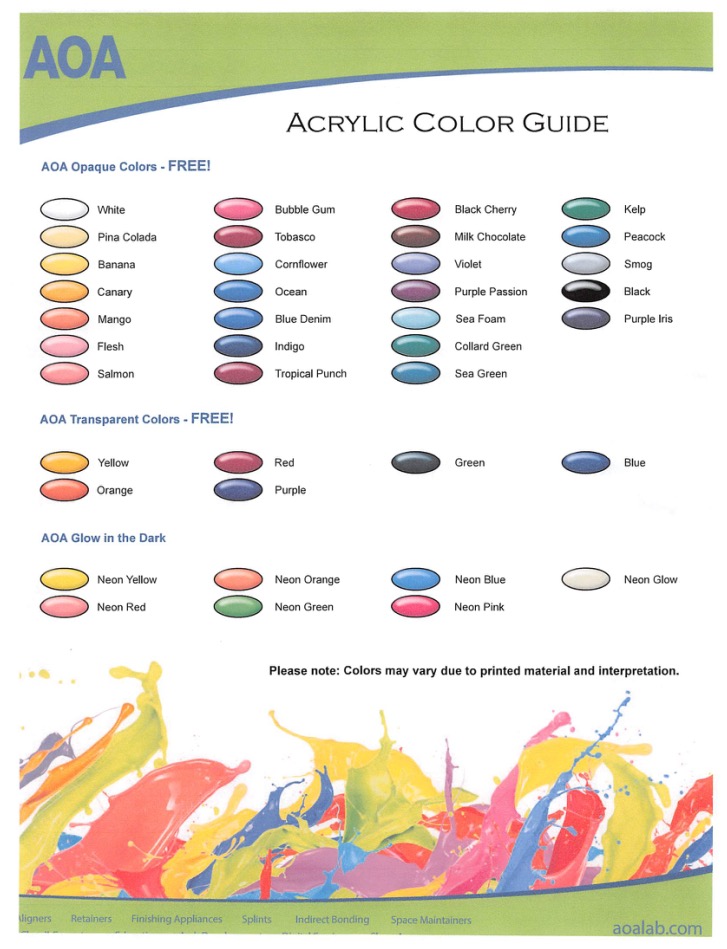This poster serves as a comprehensive paint guide for AOA's acrylic color range. Dominating the top section is a striking splash of green paint, across which "AOA" is written in bold, blue-gray capital letters on the left side. Below, "Acrylic Color Guide" is elegantly printed in a brown-black font. A blue-gray curved line borders this green section at the bottom, adding to the colorful layout.

The guide is methodically divided into three main sections: AOA Opaque Colors, AOA Transparent Colors, and AOA Glow in the Dark Colors, each denoted as "FREE!" in capital letters using the same blue-gray font. Each section features rows of oval color swatches, resembling jelly beans, each paired with its corresponding name. In the AOA Opaque Colors, hues range from whites and pastels like "Pina Colada" and "Banana" to vibrant colors like "Tabasco" and "Peacock." The AOA Transparent Colors include standard shades such as yellow, orange, red, purple, green, and blue. Meanwhile, the AOA Glow in the Dark Colors feature neon shades such as neon yellow, neon red, neon orange, neon green, neon blue, neon pink, and neon glow.

At the bottom of the poster, there’s a disclaimer in black font: "Please note colors may vary due to printed material and interpretation." Adding to the artistic flair, the lower section displays an abstract splash of vivid colors, including yellow, orange, pink, light blue, and purple, along with additional green swatches and an unreadable footnote. On the far right, the poster concludes with "AOALAB.com" in the same blue-gray font.